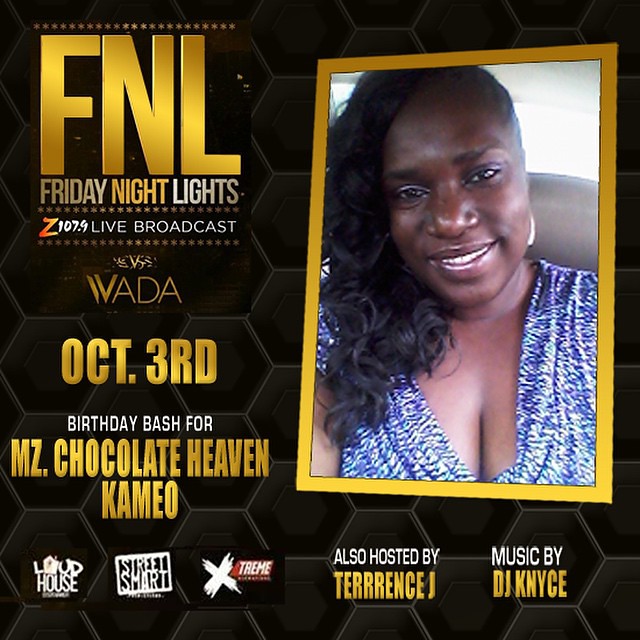The image is a promotional poster with a sleek black background adorned with a light gray honeycomb pattern. Occupying the top left corner in bold, gold letters is the acronym "FNL," followed by "Friday Night Lights" in smaller gold text, and "Z107.9 Live Broadcast" in white. Just below, "WADA" is inscribed in white, leading to a crucial event detail in bold gold text: "October 3rd." This event is a "Birthday Bash for MZ Chocolate Heaven Cameo."

Prominently on the right side is a photograph of a smiling black woman with her hair elegantly parted to one side. She is wearing a blue shirt, and the photo is encased in a gold border, giving it a regal touch. Beneath this, a list of sponsor names appears: "Loud House," "Street Smart," and "Xtreme."

At the bottom, additional event information is included in white and gold text: "Also hosted by Terrence J," and "Music by DJ Nice."